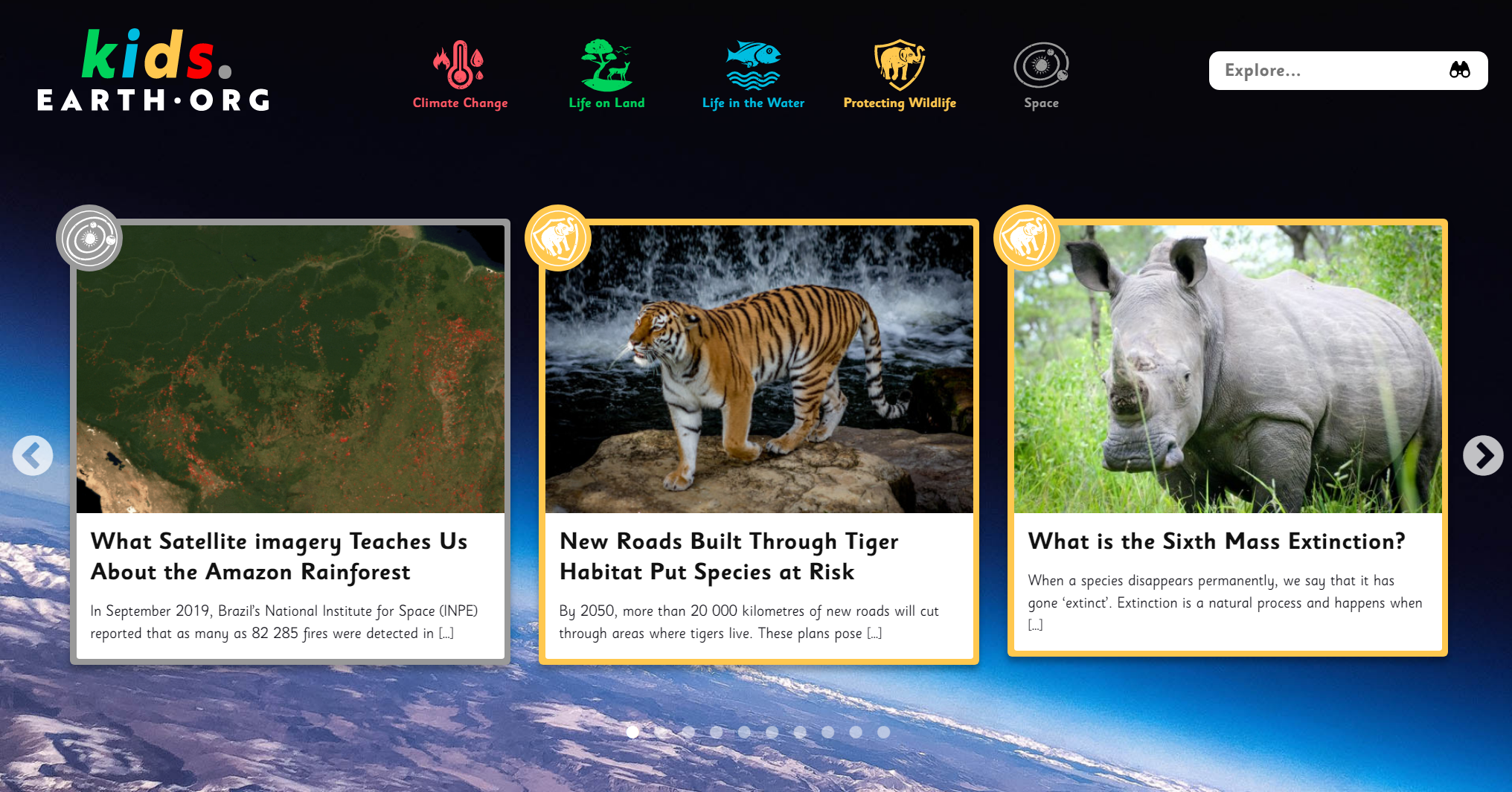The website appears to be a vibrant educational platform designed for children to learn about Earth and Earth sciences, featuring a captivating outer space theme. The background image prominently displays a breathtaking view of our planet from space. The top half of the image is dominated by the black expanse of space, while the lower right portion showcases the majestic curve of Earth, with the atmosphere glowing faintly above. The planet's horizon and atmospheric line are set at a gentle diagonal, rising from the lower right corner towards the top left, but not connecting directly with either corner.

The website's title, "kids.earth.org," is creatively rendered with the word "kids" in colorful letters: K in green, I in blue, D in yellow, and S in red. The remaining portion, ".earth.org," is in more subdued tones, with the dots appearing grey and the words in white.

Across the top of the homepage, there are several navigational choices, each with distinctive icons:
- "Climate Change" in red, accompanied by a thermometer icon.
- "Life on Land" in green, illustrated with an image of a giraffe standing under a tree.
- "Life in the Water" in blue, marked by a fish icon.
- "Protecting Wildlife" in yellow, symbolized by a shield surrounding an elephant.
- "Space" in green, represented by a space exploration icon.

In the top right corner, there is a convenient explorer search bar, allowing users to easily find specific content.

The website also features three highlighted articles for kids to explore:
1. A space-themed article titled "Satellite Imagery Teaches Us About the Amazon Rainforest," indicated by the space icon.
2. An article under "Protecting Wildlife" discussing the risks posed by new roads built through tiger habitats titled "New Roads Built Through Tiger Habitat Put Species at Risk."
3. Another "Protecting Wildlife" article on "What is the Sixth Mass Extinction."

With its engaging visuals and diverse educational topics, this website is a rich resource for young learners eager to discover more about our planet and the various environmental issues it faces.